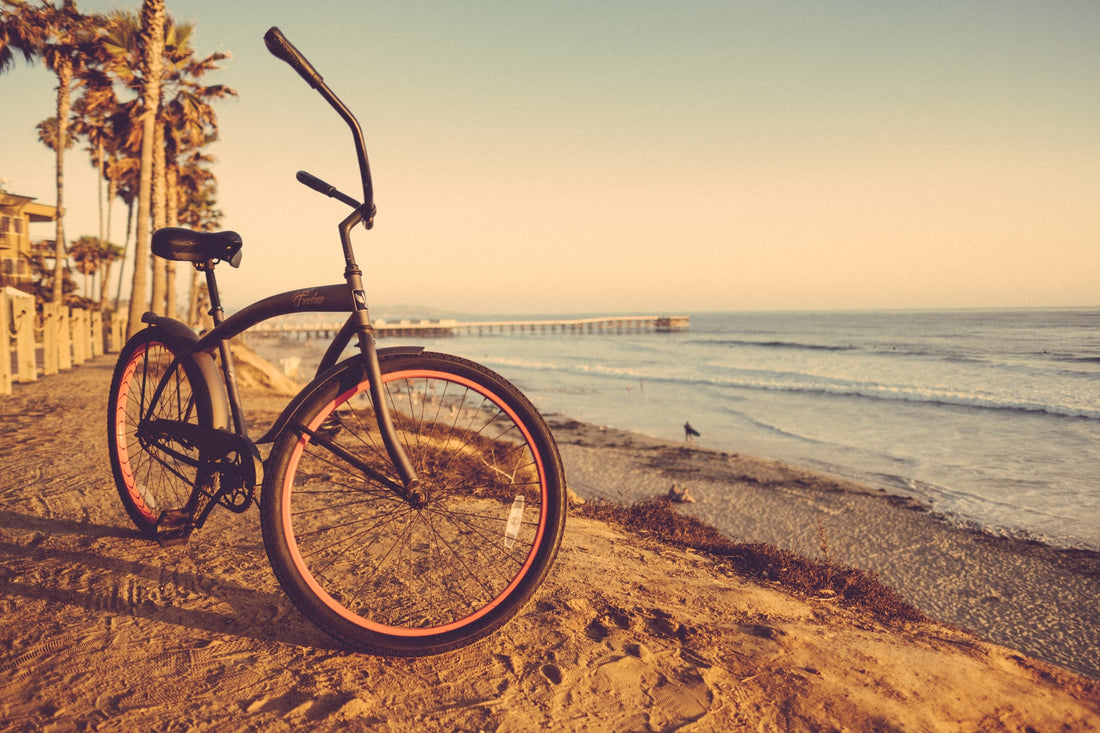The photograph captures a serene beach scene with a calm shoreline, featuring a black bicycle with dark orange or light red-rimmed tires parked on a strip of soft sand. The setting sun casts a gentle shadow on the bike, hinting at the golden hour. In the background, several palm trees line the beach, adding a tropical feel to the image. A white and brown pier extends into the tranquil water, creating a picturesque backdrop. To the left of the bicycle, there is a wooden rope fence and the partial view of a building. The scene appears to have a filtered, possibly sepia, effect, enhancing the warm, nostalgic atmosphere, and a bird can be seen nearby on the shoreline.